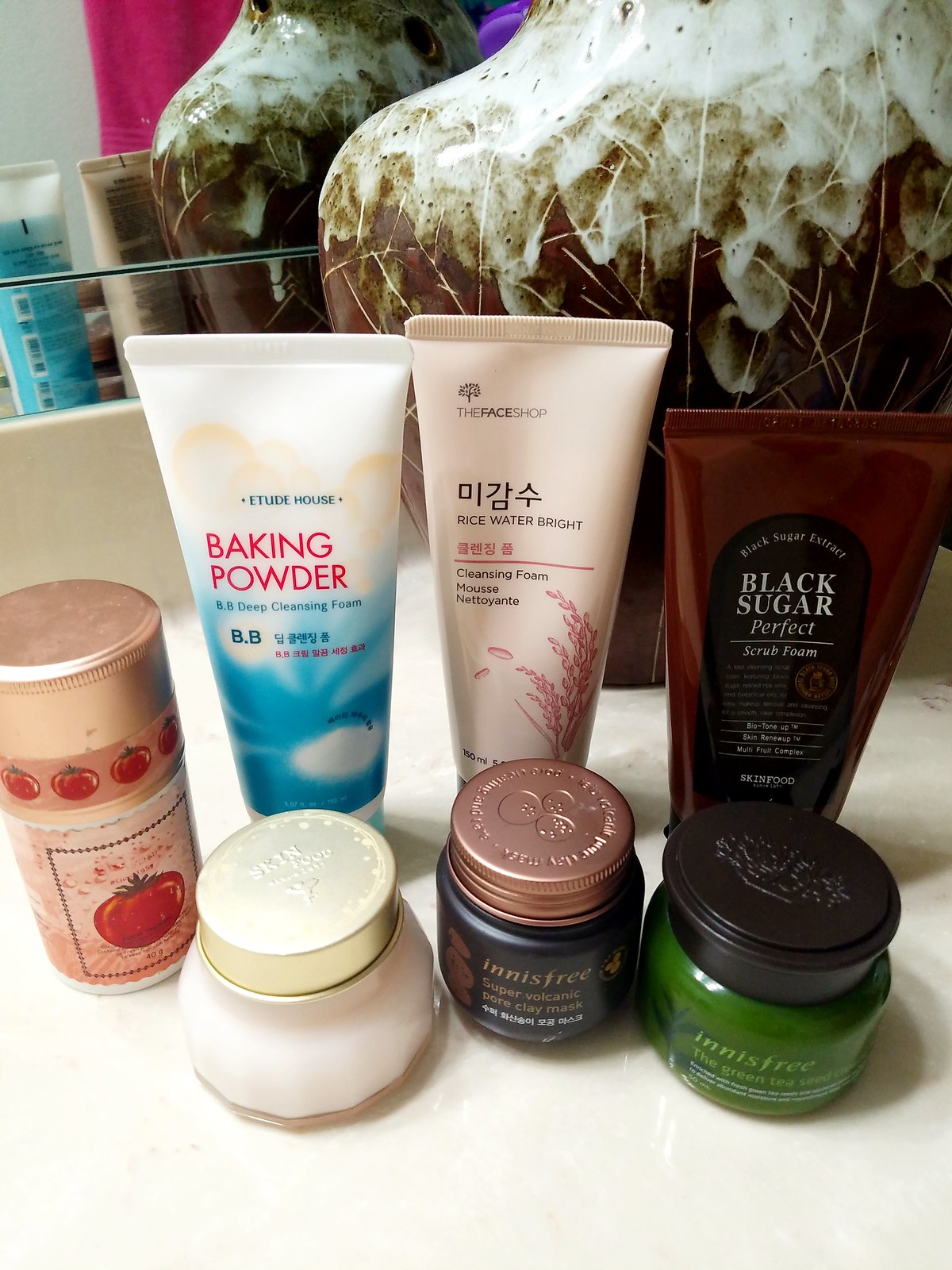**Detailed Caption for Image of Beauty Products:**

This image showcases an array of seven beauty products neatly arranged on a marble countertop, which is likely in a bathroom setting given the matching marble backsplash and a large mirror in the background. A large, eye-catching brown and white vase or statue dominates the rear of the scene, contributing to the decor. The mirror, however, has a noticeable line or crack at the bottom portion.

**Products:**
From left to right, the products are as follows:

1. **Tall Can with Tomatoes:**
   - **Description:** This is the tallest can among the group. It features a golden jar top design with a label adorned with a continuous pattern of small tomatoes. The lower part of the label is pinkish with diamond-shaped motifs, each centered with a small tomato.
   
2. **Gold-Capped Jar (Skin Food):** 
   - **Description:** Positioned in front of the tomato can, this jar has a gold cover and bears the words "Skin Food," accompanied by a small emblem that appears to be a cherub. The jar itself is either white or pink, potentially clear, showcasing the product inside, which gives it a scalloped appearance.
   
3. **Innisfree Volcanic Mask:**
   - **Description:** This is a black jar with a brownish lid. The top of the jar reads "Volcanic," and the side label says "Innisfree" in gold lettering. Below that, it states "Super Volcanic Pore Clay Mask" along with some Asian script. The design includes a logo with three circles resembling a snowman.
   
4. **Innisfree Green Tea Seed Jar:**
   - **Description:** This green jar has a lid embossed with a branch or tree design. It’s labeled "Innisfree" and also features "Green Tea Seed" among other text, which is partially obscured. There is also a small plant graphic near the words.
   
5. **Etude House Baking Powder Tube:**
   - **Description:** The first of the trio of squeeze tubes in the back. It is white with a blue label for "Etude House" and red "Baking Powder." The product is described as "BB Deep Cleansing Foam" with accompanying Asian characters. The design features a gradient blue-to-white background and gold circles.
   
6. **The Face Shop Rice Water Bright Tube:**
   - **Description:** This pale pink or off-white tube features a tree logo and "The Face Shop" branding, followed by "Rice Water Bright." Additional text includes Asian characters and "Cleansing Foam Mousse," with a willow branch illustration and measurement details of 150 ml.
   
7. **Skin Food Black Sugar Perfect Scrub Foam Tube:**
   - **Description:** The final product is a brown squeeze tube with a black label and half-circle top. It states "Black Sugar Extract, Black Sugar Perfect" followed by "Scrub Foam." Several lines of text are too blurry to distinguish, but it also includes a gold logo and mentions "Skin Renew," "Multi-Fruit Complex," and is branded as "Skin Food."

These detailed descriptions bring into focus the diverse range of beauty products featured in the image, each with its distinctive packaging and branding.